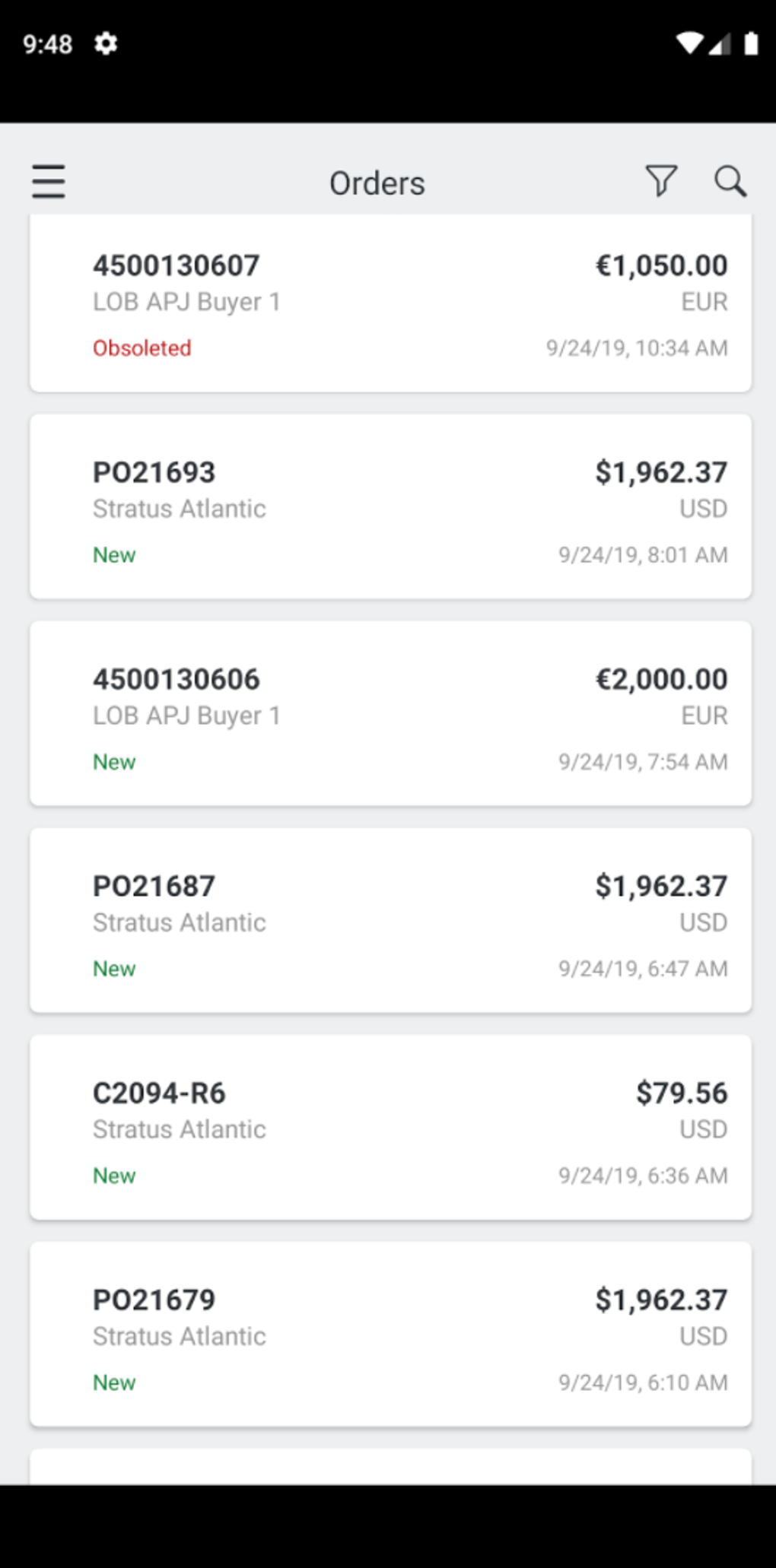This image showcases a detailed screenshot of a website on a cell phone, highlighting various elements and information. 

At the top, a horizontal black bar runs across the screen. On the left-hand side of this bar, the time "9:48" is displayed in white. Right beside it, there's a Settings button icon. Moving towards the right of the bar, signal strength bars, a Wi-Fi icon, and a full battery icon are sequentially displayed.

Below this, on the left, there are three vertically aligned black lines, likely indicating a menu. Centrally located, the word "Orders" is displayed prominently. To the right, there is a black key icon, and further to the right is a magnifying glass icon, representing a search function.

Further down, a section begins with the text "A500-130607" on the left, paired with "1,050 pounds EUR" on the right. Below this, "LOB APJ Fire 1" is mentioned on the left, marked as "Obsoleted" in red, indicating a non-active or phased-out item. On the bottom right of this area, the date and time "9-24-19, 10:34 AM" is displayed.

Continuing downwards, another horizontal white box appears:
- "P02-1693" is written in bold black letters at the top. 
- Below it, "Stratus Atlantic" is noted in gray letters.
- The word "New" is highlighted in green letters beneath that.
- To the right, the price "$1,962.37" is displayed in bold, and "USD" is written below it. 
- At the bottom, to the right, "9-24-19, 8:01 AM" is shown.

Further down on the left, the sequence "4500-130606" appears in bold black numbers. Below this, "LOB APJ Fire 1" is written in gray. The word "New" appears again in green letters. To the right in this section:
- "2,000 pounds" is displayed.
- Below this price, "EUR" is noted in gray.
- At the bottom, the date and time "9-24-19, 7:54 AM" is shown in gray, completing the detailed documentation of entries on the screenshot.

This refined and comprehensive description captures the intricate details of the elements shown in the cell phone website screenshot.